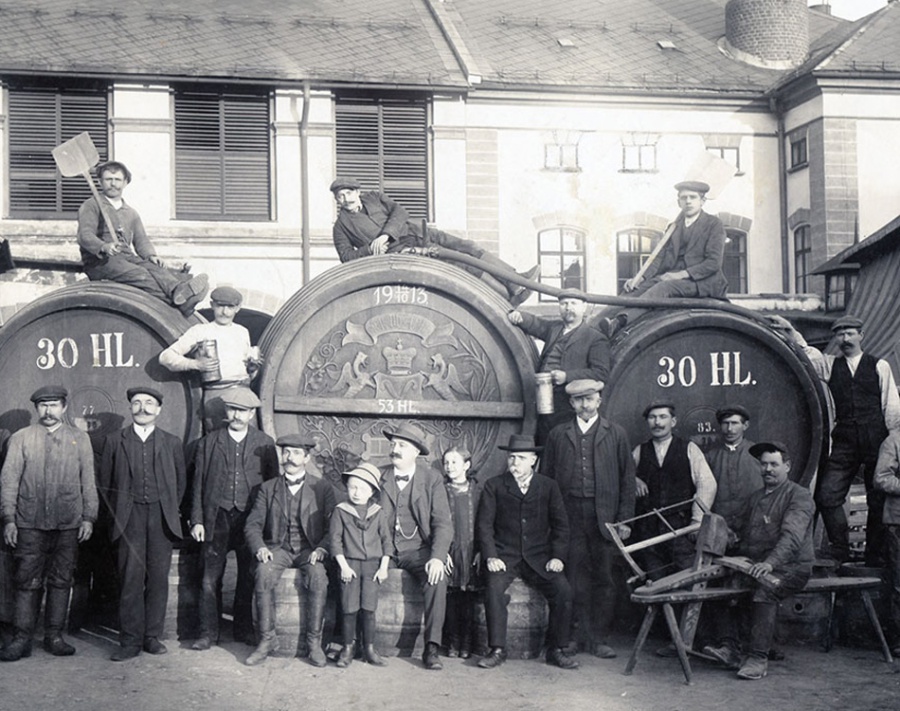This vintage black-and-white photograph, captured in either the late 1800s or very early 1900s, depicts a group of workers and a few children gathered in front of what appears to be a Czech brewery. Prominently featuring three massive wooden brewing barrels arranged horizontally from left to right, the barrels are inscribed with white text: "30 HL" on the left and right barrels, and "53 HL" with the year "1913" on the central barrel. Artistic engravings adorn the central barrel, including a shield flanked by two griffins, a crown above, and decorative vines and flowers.

The men in the imagery are posed with tools suggestive of their labor. The individual atop the left barrel sits with crossed legs, gazing directly at the camera while holding a shovel slung over his shoulder. The central figure reclines casually, supported on his elbow, wearing a hat while looking at the viewer. Meanwhile, the man on the right faces the center, brandishing a pickaxe over his shoulder, attired in a beret and jacket. Below, a wide array of workers align in front of the barrels, many sporting hats, handlebar mustaches, and traditional work attire. A distinguishable man in a bow tie sits between two children; one child to his left dons a hat, while the slightly older child without a hat sits to his right. To the right edge of the image, a man seated on a workbench holds an item in his lap and a stein in his right hand.

Behind the assembly stretches a stucco-colored building with black-trimmed windows and a gray roof, extending across the entire frame. The photo captures a slice of life from a bygone era, showcasing the workers' camaraderie and the daily grit of early 20th-century brewery life in Prague.